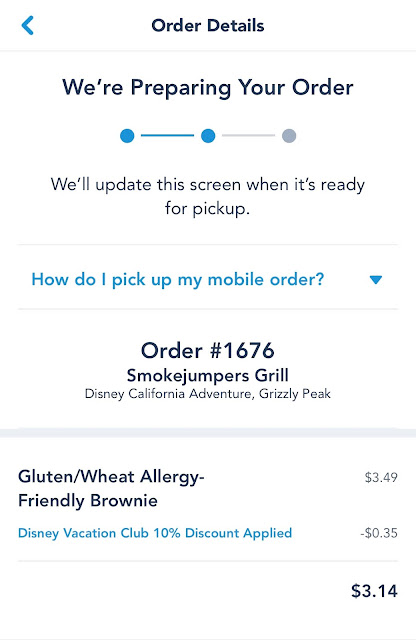This is a detailed screenshot from what appears to be a mobile device, showcasing an order preparation screen. The screenshot, oriented vertically, does not display any typical mobile status indicators like cell provider, time, or battery percentage, suggesting it focuses solely on the app's interface.

At the very top, there's a "back" arrow, indicating the user has navigated forward in the ordering process. The heading "Order Details" is prominently displayed in centered text. Right below, the phrase "We're preparing your order" reassures the user that their order is being processed. A visual progress indicator shows that they are on step 2 of 3 in the order preparation.

Following this, a centered message explains, "We'll update the screen when it's ready for pickup," providing further instructions. Below this, in blue text, the user can find an interactive chevron with the question, "How do I pick up a mobile order?" suggesting additional information is available upon tapping.

Proceeding downwards, in the largest black font on the screen, the order number "1676" is displayed, along with the eatery’s name, "Smokejumpers Grill." Smaller text beneath identifies the location as "Disney California Adventure, Grizzly Peak."

A gray separator divides this section from the itemized order. The screen lists a "Gluten/Wheat Allergy-Friendly Brownie" priced at $3.49. Below, in blue text, it's noted "Disney Vacation Club, 10% discount applied," showing a deduction of 35 cents.

Finally, the "grand total" is displayed at the lower right corner of the screen, amounting to $3.14. This concise yet comprehensive interface provides all necessary details for the user’s current order status on their mobile device.